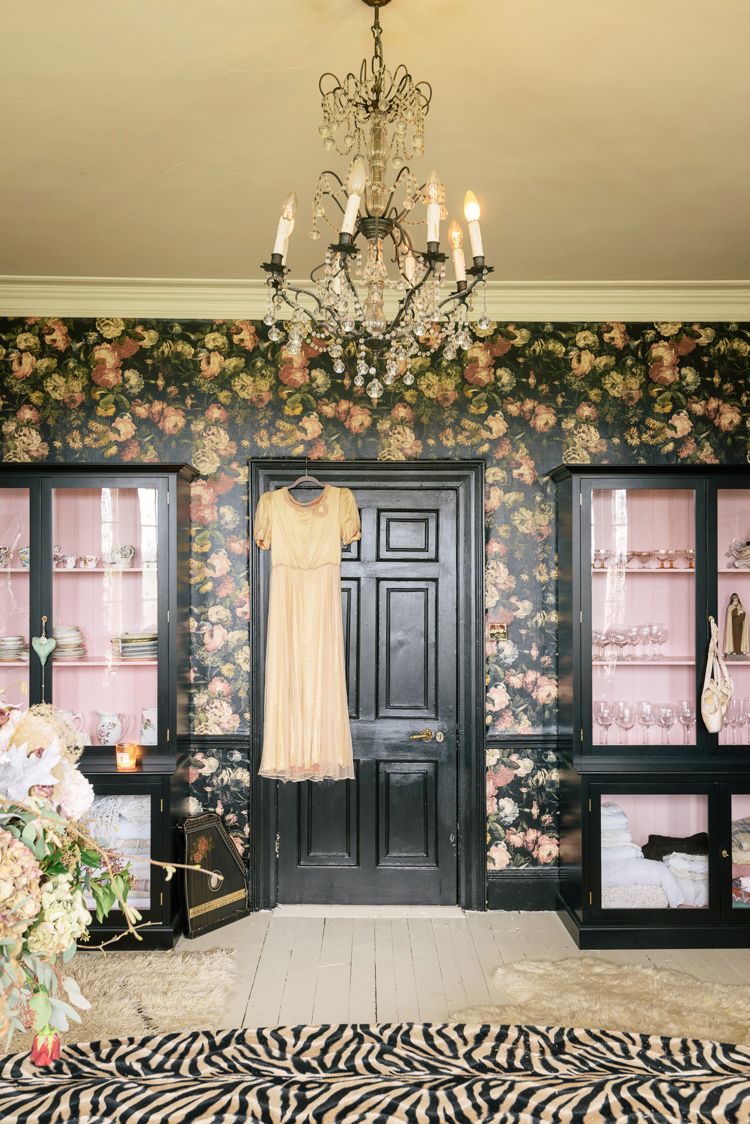The image captures a lavishly decorated room, centering on a black wooden door adorned with a long, off-white dress on a hanger. The door is positioned against a wall covered in black wallpaper with dense, colorful floral patterns, featuring shades of pink, white, red, and green. Flanking the door are two black china hutches with see-through glass doors, allowing a glimpse of neatly arranged dishes, glassware, and white linens. Inside the cabinets, the back panels are lined with pink wallpaper, enhancing the display of the items.

On the floor, there is a mix of white tiles and three distinct rugs: two are white and furry, and one features a striking zebra print extending across the lower edge of the photograph. Crown molding caps the wall with an off-white ceiling above, from which a grand chandelier adorned with hanging crystals and candle-like bulbs is suspended. To the left side of the image, partially visible in the foreground, is a lush plant adding a touch of greenery to the ornate setting.